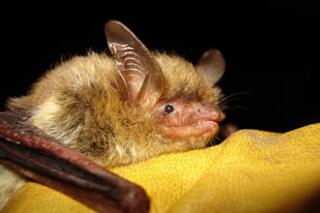This image features a bat as the central subject, set against a black backdrop. The bat is resting on a yellow surface that might be a piece of fruit or a similar object. The bat is facing to the right, showcasing its large, pointy ears, which appear tan and display visible ridges. The bat's fur is bushy and brown, lighter at the top and darker around the ears. Its face is mostly fur-less, with a peach-pink skin tone, a slightly pointed mouth, and slivers of visible teeth. The bat's black, beady eyes stand out against its pink face. The front right leg, also visible, is brown and black, featuring a horizontal black mark, and lacks fur.